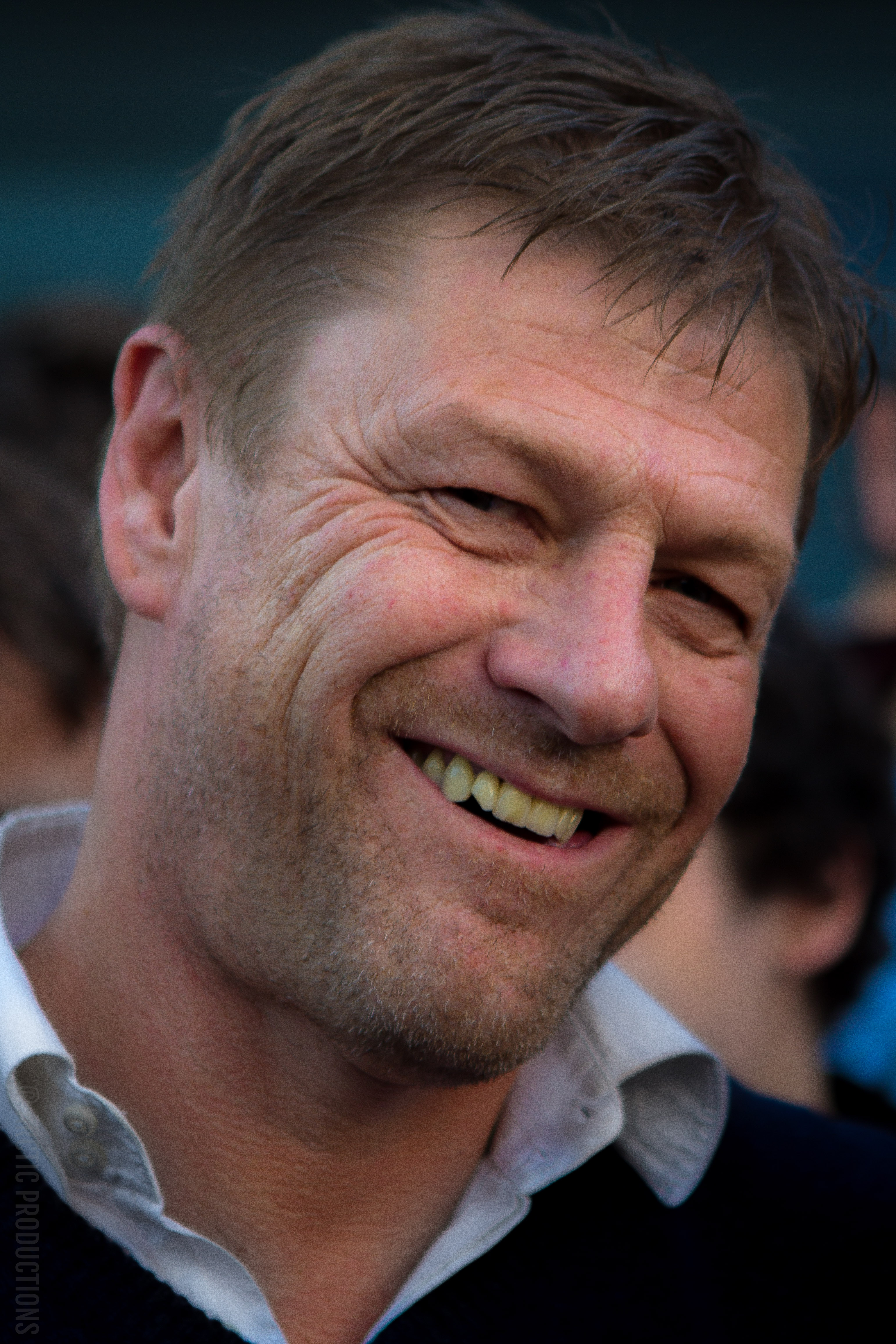The photograph features a man who appears to be in his late 40s or early 50s, smiling warmly at the camera with a broad smile that reveals his slightly stained top teeth, including a chipped tooth next to the front teeth. His short brown hair is slightly messy and combed to the side, and he has a bit of facial stubble. Wrinkles are visible on his forehead and around his squinting eyes, which look dark. His fair skin contrasts with his light blue or white button-up shirt, over which he wears a dark sweater, possibly black or navy blue. The man’s head is tilted slightly to the right. In the background, which is blurry and out of focus, other people’s heads are visible along with what seems to be dark or blue structures, perhaps bleachers.